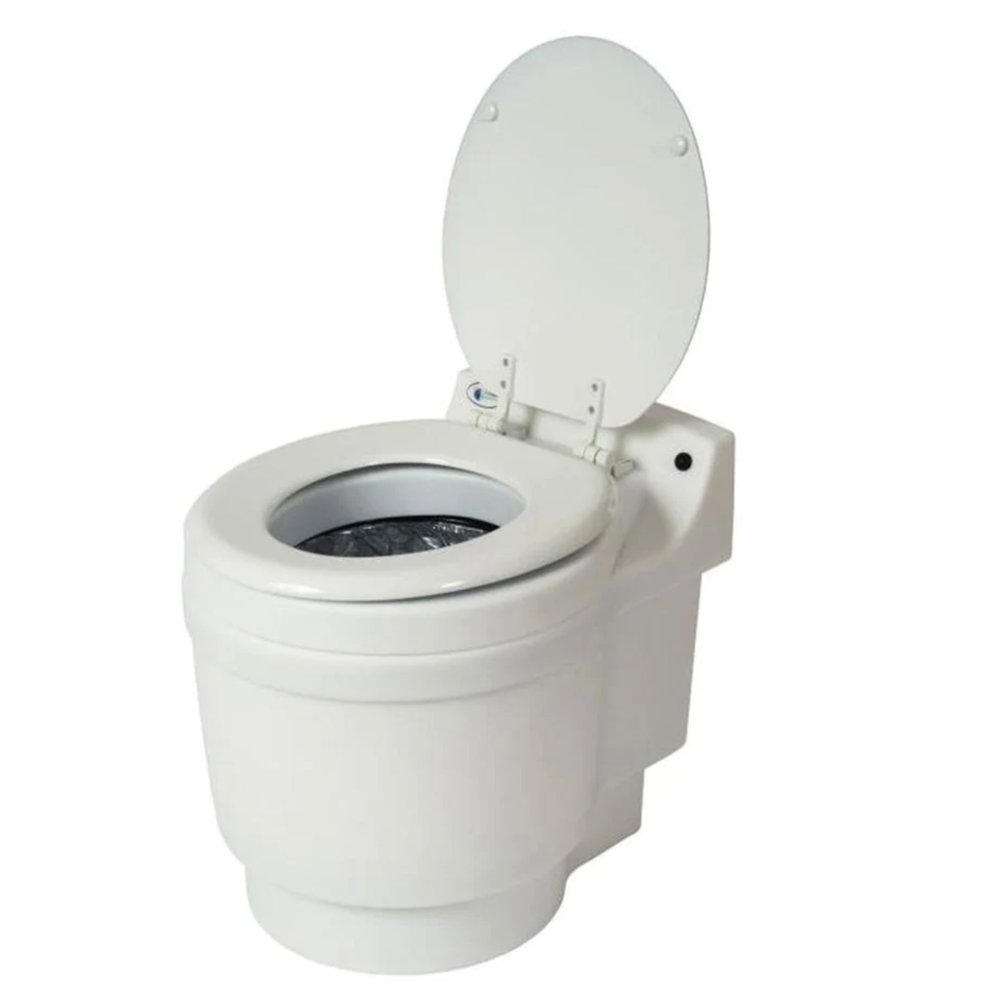The image features a large, high-tech portable toilet, set against a completely white background. The orientation of the toilet places the front side at the bottom left and the back at the upper right of the picture. The toilet seat lid is lifted, revealing the inside, which contains a black bag or surface. The white toilet has a base that resembles a white bucket with a dark marble look on the very bottom. A small hole is visible on the back behind the lid, likely for mounting something. The rim behind the toilet seat has a small logo on the left and a noticeable black button on the right. The entire composition suggests that this is a product example image, possibly for packaging or a website, showcasing the toilet's clean and modern design.